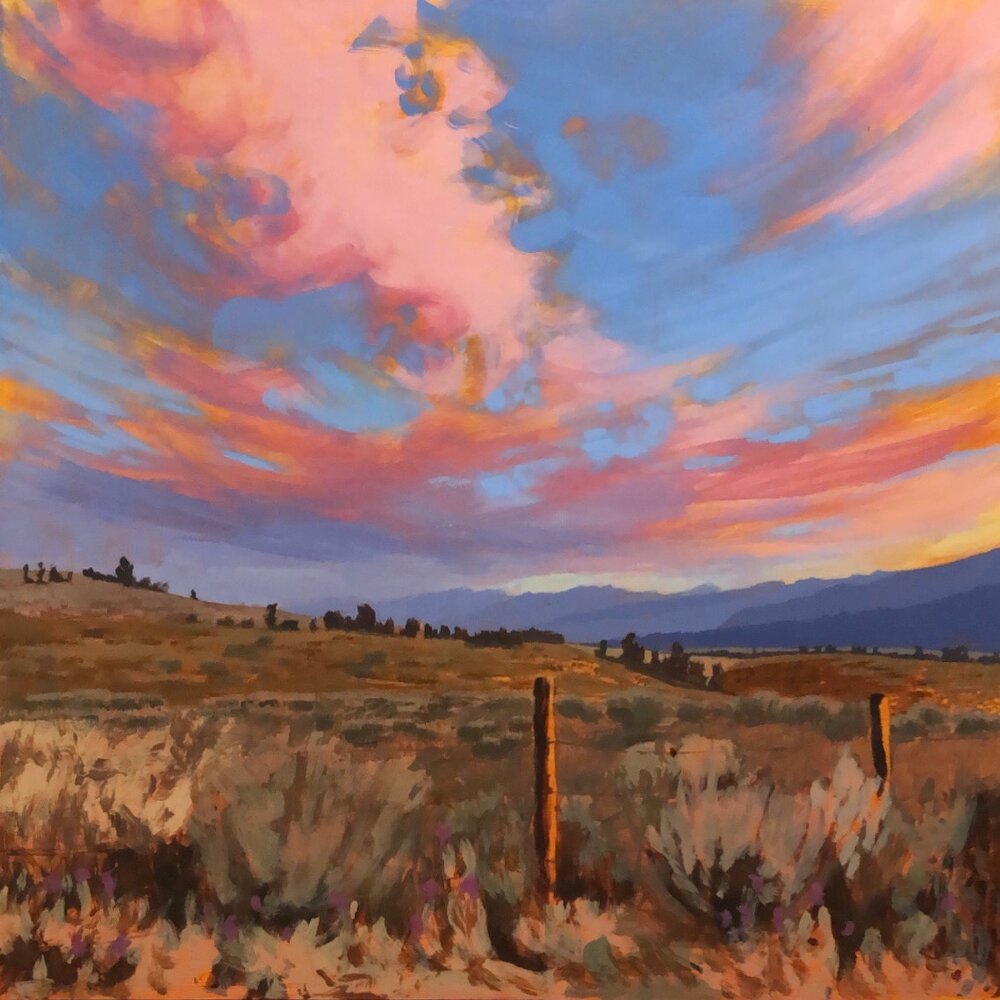The painting is a vivid depiction of a pastoral scene, likely created with oil paints or pastels, showcasing an expansive landscape. Dominating the top half of the painting is a striking sky painted in varying shades of blue, adorned with dynamic clouds that blend hues of pink, orange, purple, white, and touches of yellow, perhaps reflecting the setting or rising sun. The clouds have been rendered with a swishing motion, giving them a sense of movement, almost as if viewed through a fisheye lens.

Below the sky, the midsection of the painting features undulating hills and distant mountains. The mountains, painted in a bluish-gray, loom in the background with a rugged, craggy texture. The foreground displays a more immediate view of grassy hills and scattered vegetation. Most of the grass is brown, suggesting a fall setting or a dry season, with some green patches indicating lingering vitality or impending drought.

Two brown wooden stakes, likely part of a rough fence or gate, emerge from the ground in the forefront, accompanied by larger bushes and small, sparse greenery, adding to the rustic charm of the scene. The distinctive contrast of colors and elements in this painting creates a captivating portrayal of nature’s beauty, framed within a rural and arid environment.